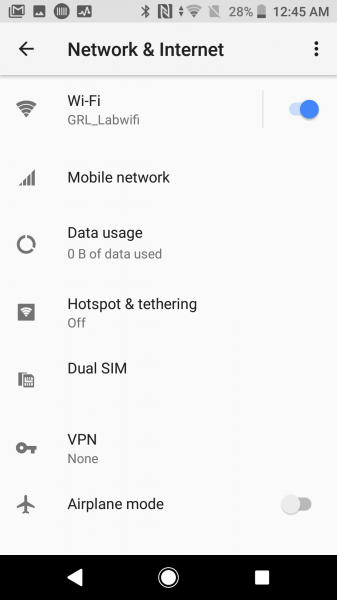This image shows a cell phone screen at 12:45 a.m. with a battery level at 28% and a weak network connection. At the top of the screen, large black text reads "Network & Internet," with a back arrow on the left and three vertically aligned dots on the right. Below this, several categories are listed with their corresponding icons:

1. **Wi-Fi**: Connected to "GRL_LAB Wi-Fi," indicated by an icon and a blue circle on the right.
2. **Mobile Network**: Details not expanded.
3. **Data Usage**: Details not expanded.
4. **Hotspot & Tethering**: Listed as "Off."
5. **Dual SIM**: Label present, but no additional information.
6. **VPN**: Displayed as "None."
7. **Airplane Mode**: Represented by an airplane icon on the left with a slider set to "Off."

At the bottom of the screen, there's a white home button in the center, a white back arrow on the left, and a white square (overview button) on the right.